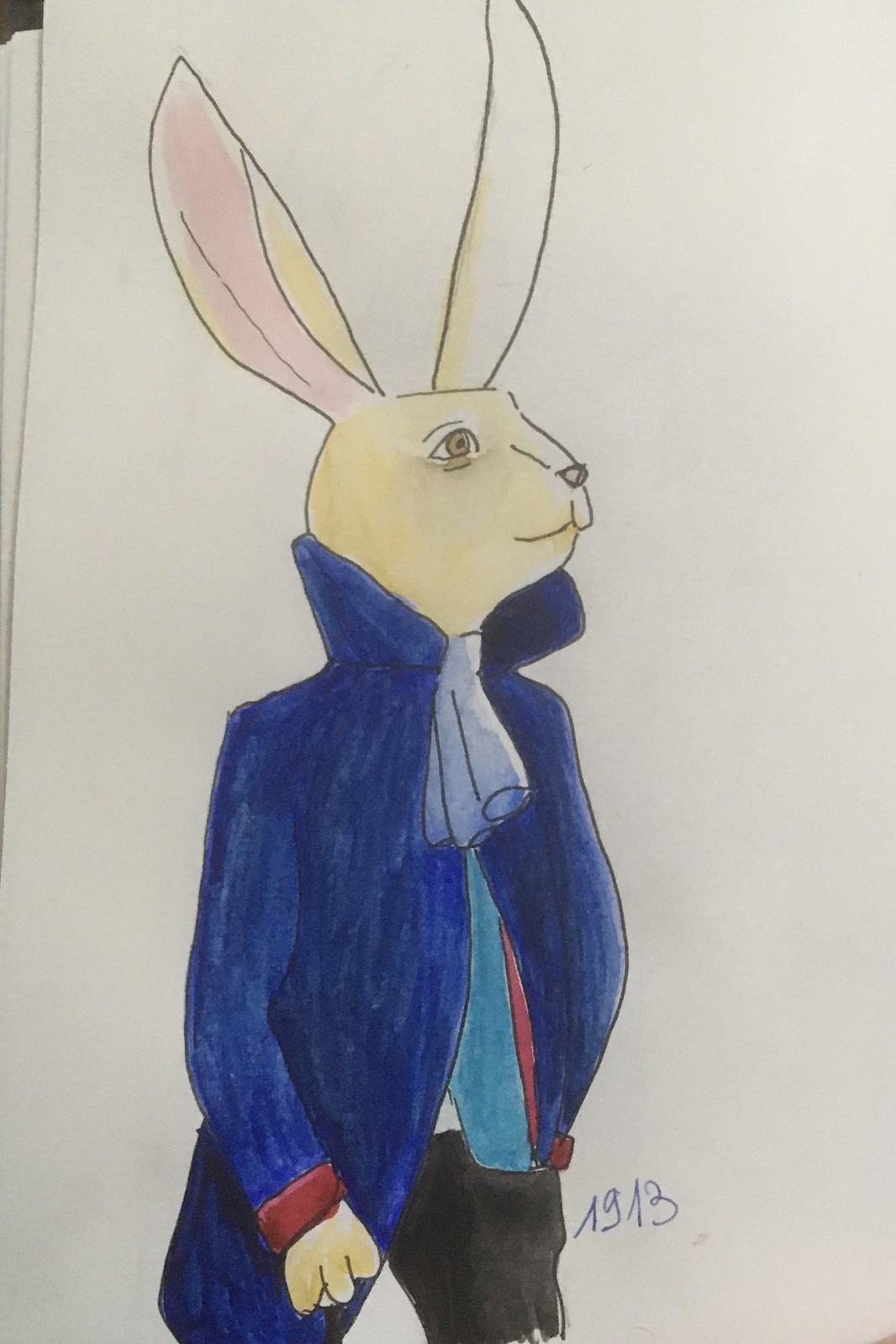This is a drawing rendered with markers on a long, white sheet of paper. It features a white rabbit with somewhat humanized facial features. The rabbit's long ears are pink on the inside; one ear stands erect while the other is slightly turned, revealing its pink interior. He is dressed in a royal blue jacket with the collar turned up, layered over a white blouse with a ruffled neck. Underneath the jacket, he wears a light blue vest and black pants. His left hand is casually placed in his pants pocket, while his right hand holds a walking stick. The rabbit has brown eyes, adding a touch of life to its whimsical, anthropomorphic appearance.